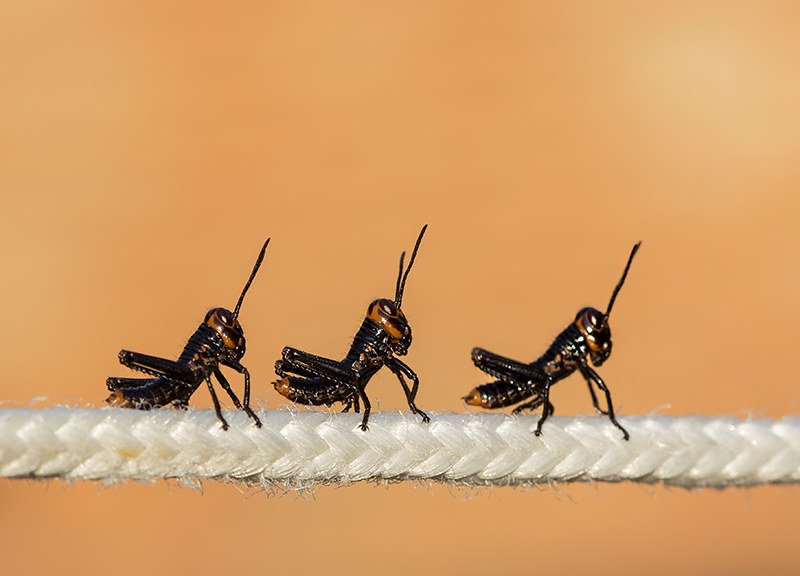This close-up photograph captures three black grasshoppers with striking orange markings on their heads, thoraxes, and abdomens, perched in a row on a white braided string. The intricate braiding of the string closely resembles rope, enhancing its textured appearance. The grasshoppers have two long, pointed antennae and appear meticulously detailed, potentially suggesting they might be intricately crafted models rather than real insects. Their legs are strategically angled as if poised to leap. The background is a vibrant orange-peach color, providing a stark contrast to the dark, glossy bodies of the grasshoppers. The overall setup presents a lifelike and intriguing composition, highlighting both the naturalistic details of the insects and the finely woven structure of the string they stand on.